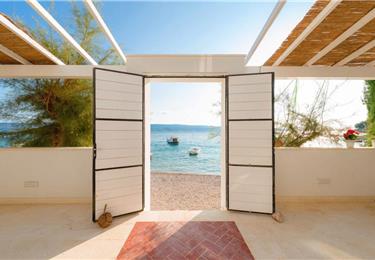This image features a bright and airy covered patio, likely part of a holiday resort, with a serene beach scene beyond. The patio has a half-height white wall and double doors made of white slats with black metal frames, creating a see-through effect. The doors, propped open by large rocks, reveal a picturesque view of sandy beach, calm blue ocean, and a couple of boats bobbing in the water. The sky is clear with a bright blue hue, meeting the horizon in the distance.

Inside the patio, on either side of the doorway, there are windows through which you can glimpse green trees and possibly a strip of grass, suggesting a lush environment beyond the sandy beach. The ceiling consists of white wooden beams interspersed with a beige straw mat, adding to the open-air, sunroom feel of the space. The floor is made of off-white stone or concrete, with red paver blocks forming a pathway leading up to the doors. A white flower pot with red flowers sits to one side, adding a dash of vibrant color to the tranquil setting.